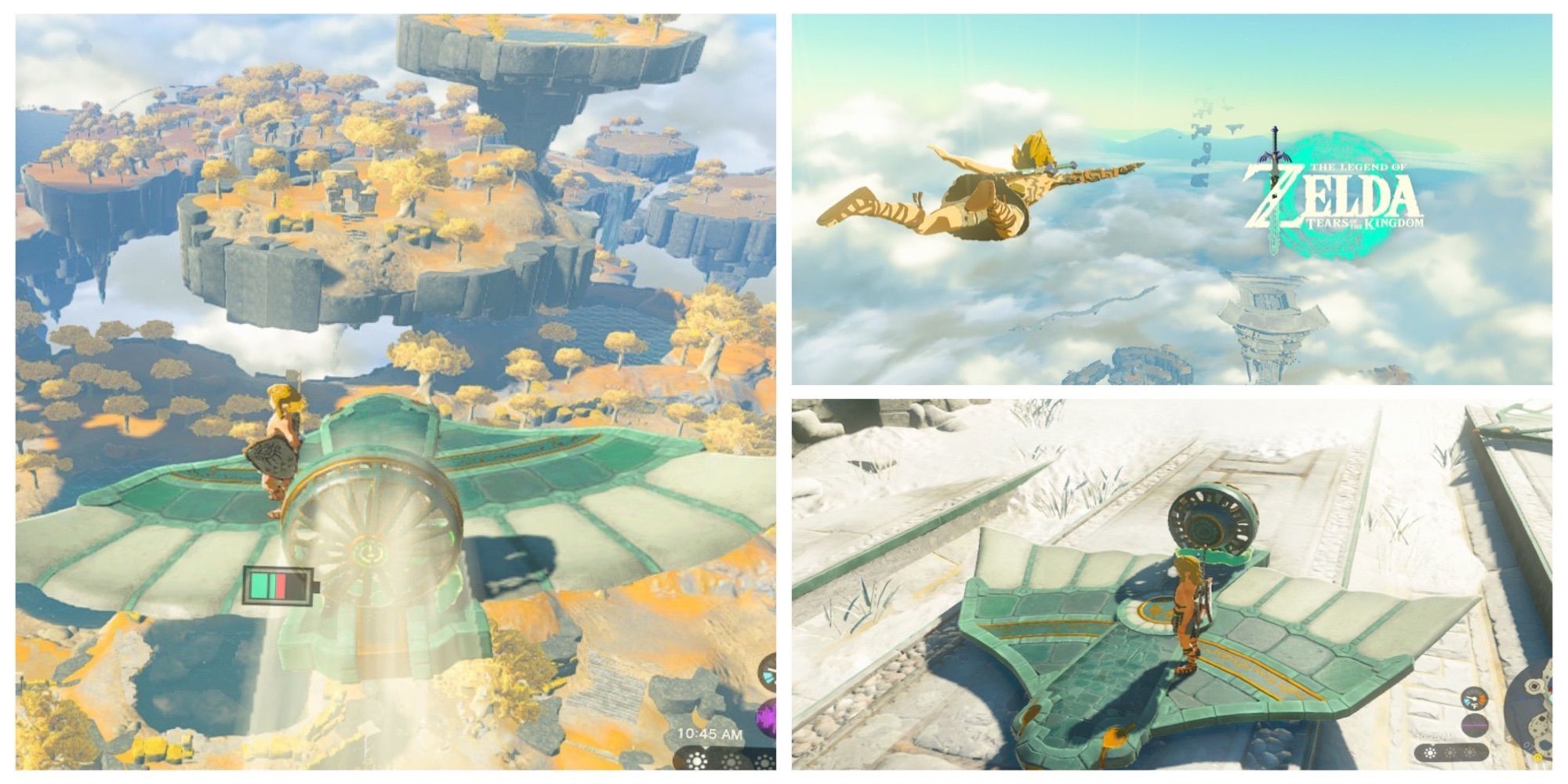This image, resembling computer-generated cartoon screenshots from a video game, is split into three panels: one large panel on the left and two smaller panels on the right. Titled "The Legend of Zelda: Tears of the Kingdom," the top right panel showcases a character with blonde hair, wearing a kilt and sandals, flying above the clouds. Next to the character is a green circle emblazoned with the word "Zelda." The bottom right panel depicts the character standing on a green and white bird-like platform, possibly a flight mechanism, situated on a ground platform within what seems to be a white temple. This platform features a battery icon indicating its power level. The large left panel displays a similar scene where the character soars on the bird-like craft over a fantastical floating kingdom with yellow grass and trees. The flying object is shown with rays emanating from its back, signifying motion.